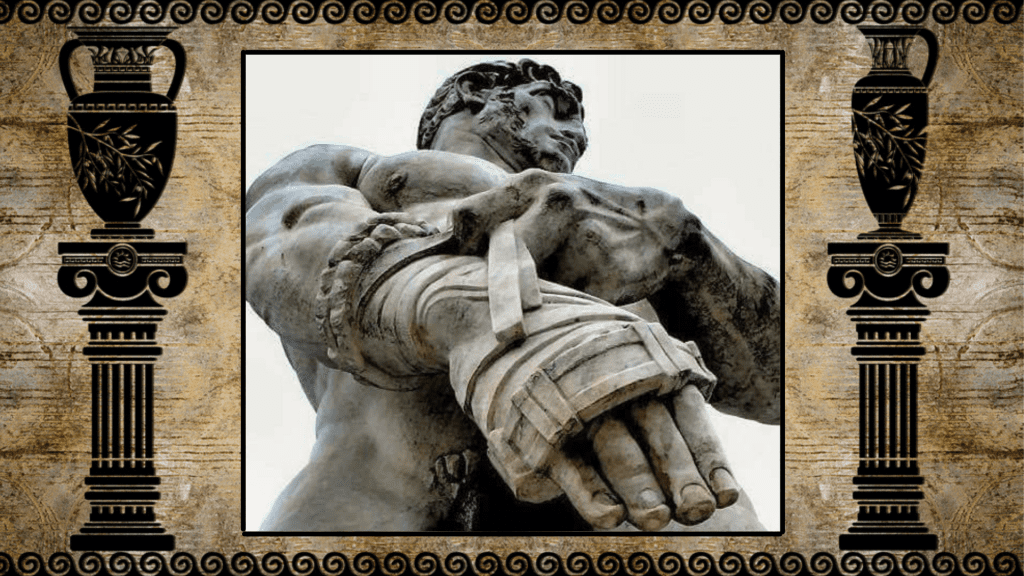This color image features a composite artwork with a two-by-one aspect ratio, wider than it is tall. The border is adorned with intricate swirly designs on the top and bottom, while the left and right sides showcase illustrations of Greek or Roman-style columns topped with urns. The urn on the left has two handles and contains flowers, whereas the urn on the right has one handle with similar floral adornments.

At the center of this elaborate frame, a square black-and-white photograph captures a striking statue. The perspective appears to be from below, accentuating the imposing nature of the figure, which closely resembles the classical 'statue of David' with its detailed curls and ridges in the hair. The figure is muscular and depicted with minimal clothing, sporting a wrapped bandage around its right arm, hinting at a boxer or warrior aesthetic. The statue's stance is dynamic; it faces forward but looks off to its left, with its left hand positioning to obscure the crotch area. The overall scene gives off a distinct aura of ancient mythology, possibly Greek, encapsulating the essence of a heroic, Olympian figure.